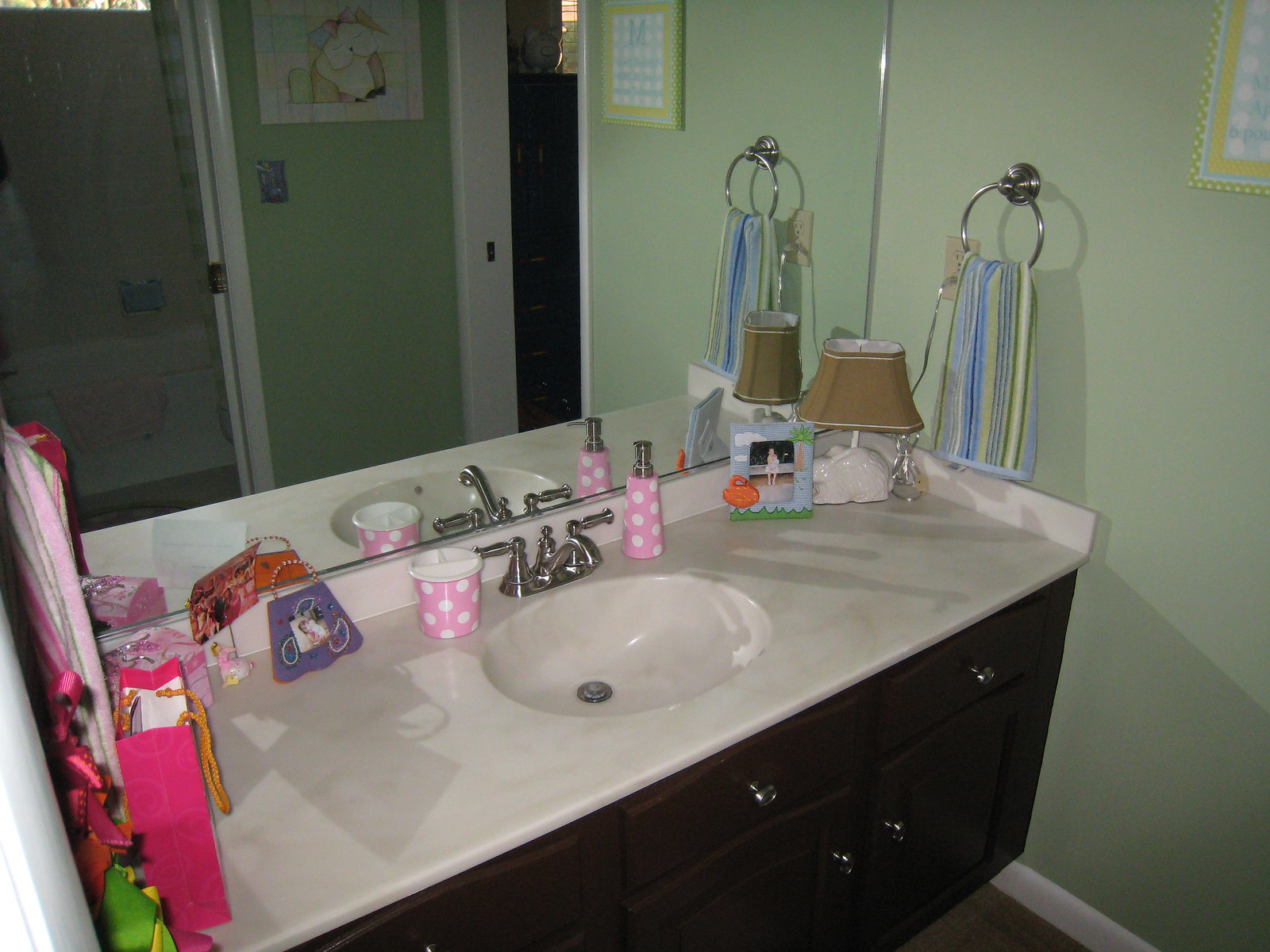This photograph depicts a bathroom setting that evokes the design sensibilities of the late 1980s and early 1990s. The vanity unit features a light-colored surface with a faint marble pattern, indicative of synthetic materials popular during that era. Integrated into the countertop is a bowl sink, which complements the period look. 

The backsplash and mirror similarly reflect the style of the late 20th century, reminiscent of those used extensively in prefab and modular homes. Contrasting with these vintage elements, a modern, updated faucet and coordinating ring towel racks, all with matching patina, suggest recent updates.

The cabinetry beneath the sink is dark, synthetic wood, again reinforcing the retro aesthetic. Chrome handles adorn the cabinet doors, adding to the nostalgic ambiance. The floor features a light-colored mop board, while the walls are painted a flat grayish-green, unifying the color scheme.

Atop the counter, a pink shopping-style gift bag stands out, accompanied by another small decorative bag. Additional items include a decorative photo holder with pink and white dots, a soap dispenser, a toothpaste holder, and a lamp with a shade situated in the right corner. Towels hang neatly on a rack to the left, completing this carefully curated bathroom scene.